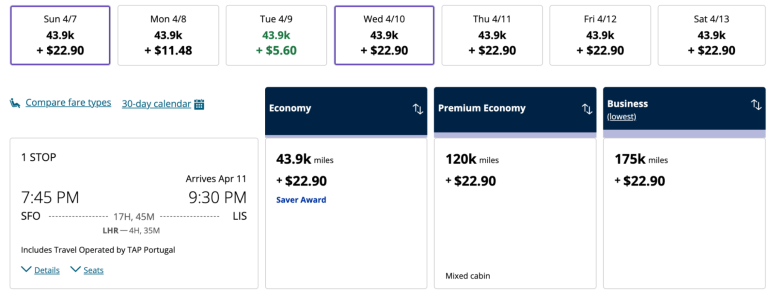The image depicts a rectangular information chart divided into sections, providing details about a travel site. The top row consists of seven squares, each representing a day of the week from Sunday through Saturday. Each square contains data on the number of thousand miles required and additional pricing details for travel on that day.

The second row features a section labeled "Compare fare types on a 30-day calendar," which spans about two and a half squares. This section is clickable, allowing users to explore different fare comparisons over a month.

Next to this, there are three squares with columns titled "Economy," "Premium Economy," and "Business," showcasing various fare classes.

Starting from the subsequent row, the chart includes a travel itinerary with a single stop. It details a flight departing at 7:45 PM and arriving at 9:30 PM on April 11th, operated by TAP Portugal. Additional blue drop-down boxes provide further details and statistics about the journey.

For this specific flight (7:45 PM to 9:30 PM with one stop), the chart lists fare options for Economy, Premium Economy, and Business classes.